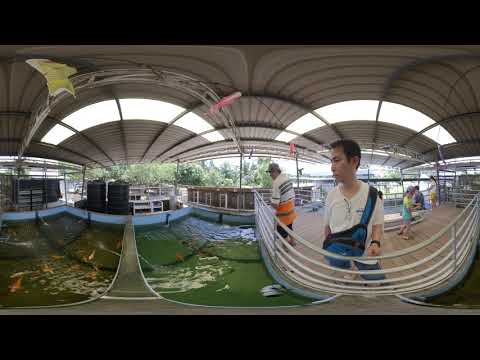The photograph captures a vibrant scene of a large indoor koi pond, bordered by a wooden boardwalk with a metal fence composed of four-foot-tall metal rods. Numerous spectators, likely in Japan given the predominantly Asian appearance of the crowd, are gathered by the railing. Notable individuals in the image include a young man in his mid-20s, closest to the camera, wearing a white t-shirt with glasses clipped to the collar and a blue, black-accented man bag slung diagonally across his torso. Next to him stands a man in an orange, gray, and white striped shirt, donning a tan baseball hat. The photograph, taken with a fisheye lens or possibly a 360-degree camera, exhibits a distinctive warping effect, providing a wide, immersive view of the area. The koi pond teems with vibrant fish, drawing the attentive gazes of the onlookers. The scene is framed by black bands at the top and bottom, adding a unique visual aspect to the image.